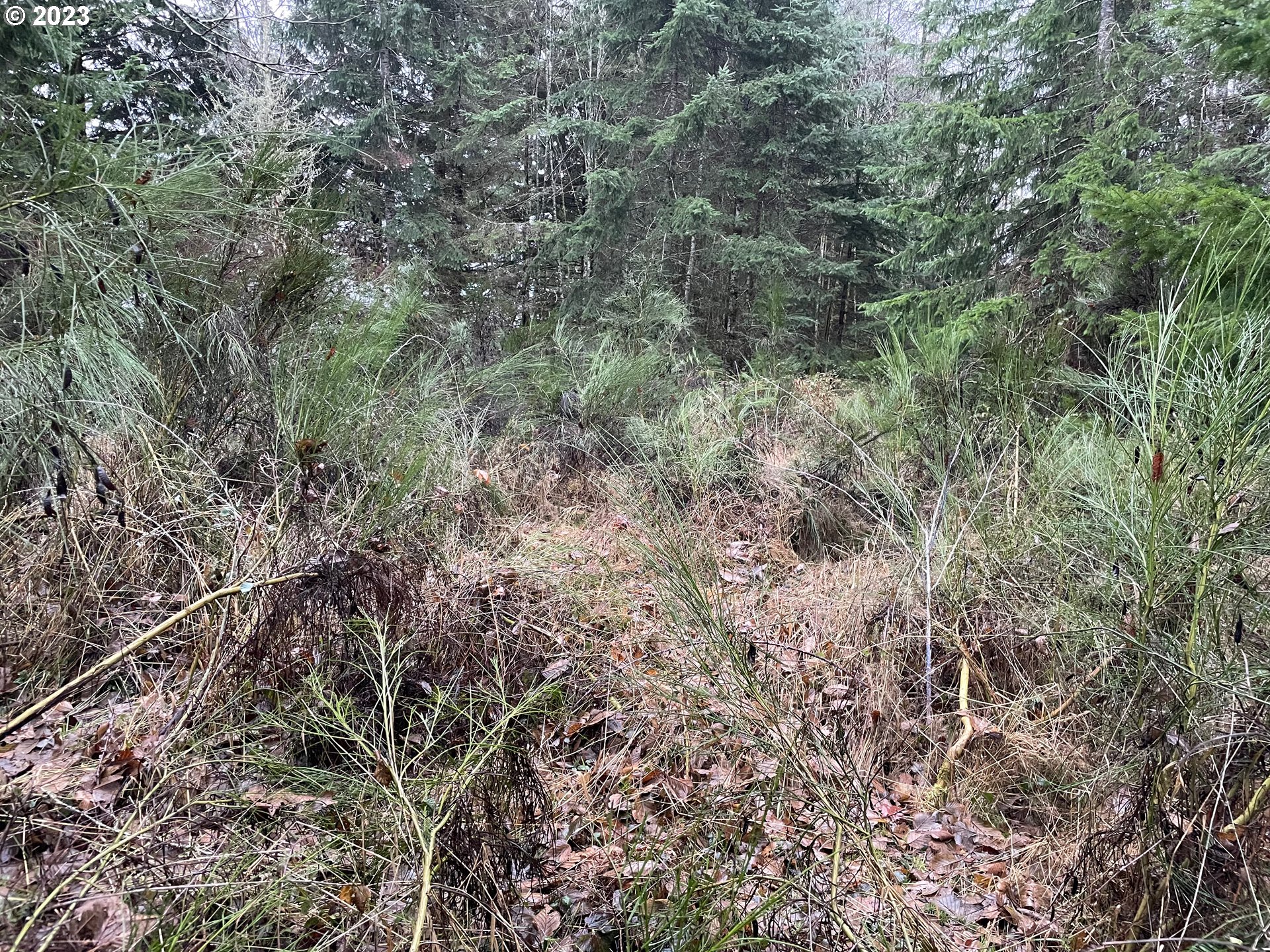This detailed color photograph captures a dense forest scene, marked by a clearing that has evidently seen significant foot traffic from both people and animals. The trail at the center is visibly trampled, showing a distinct path with patches of bare, compacted earth and dried grasses swirled around. Surrounding the path, lush, tall grasses rise to head height or more, indicating the overgrown nature of the setting. On either side of the trail, the verdant foliage and dense plant growth make traversing difficult without pushing through or cutting back branches. The forest features a mix of evergreen and deciduous trees. The evergreens, mainly young pine trees, form small clumps with closely grown trunks, while mature, towering trees populate the background. There is a slight glimpse of a gray-white overcast sky through gaps in the thick tree canopy, hinting at dim daylight. The diversity of vegetation includes green bushes, dried grass, and a thick layer of multicolored dead leaves strewn across the forest floor, which appears slightly muddy in spots, suggesting recent moisture. A subtle but notable detail in the top left corner is a light pinkish-white text stating "copyright 2023," adding an official touch to the photograph. Overall, the image vividly portrays the untamed beauty of a woodland area in the process of natural succession, with elements of both living and decaying flora.